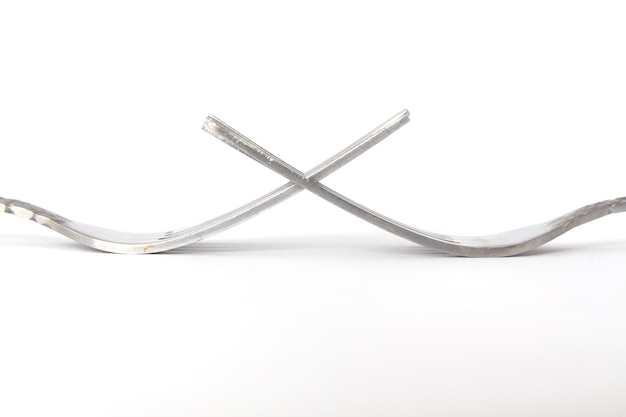This up-close color photograph showcases two silver forks intricately intertwined through their tines, forming an almost perfect X shape. The forks are positioned on a white surface against a white background, creating a minimalistic and clean aesthetic. Notable are the imperfections on the forks, such as dings and a noticeable rust stain or dirty spot on the left fork. The handles exhibit a textured pattern, adding to the visual interest. The overlapping tines create a detailed, almost bow-like, intricate shape at their intersection. The focus is solely on the forks, with no other objects, text, or organisms present in the image.